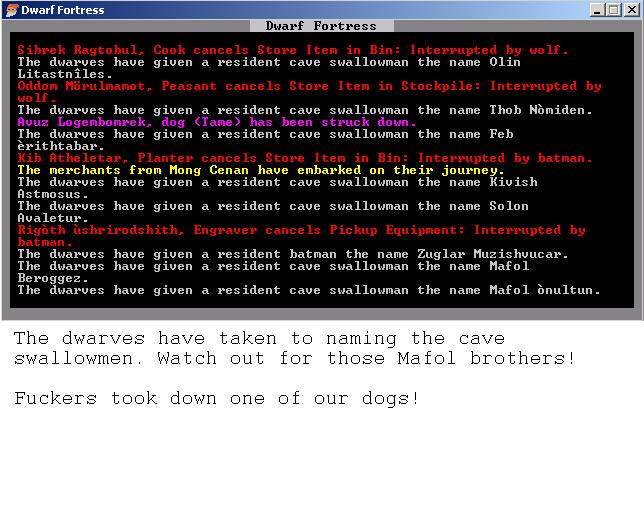The image depicts an old computer screen, reminiscent of early Windows or DOS interfaces, showcasing a screenshot from the game Dwarf Fortress. The screen is predominantly black with text displayed in various colors—red, white, purple, and yellow. At the top left corner, "Dwarf Fortress" is prominently displayed. The text includes game events such as "Dwarf Fortress, Sybrick, rag to bowl, cook, cancel, store item in bin, interrupted by a wolf" and "The dwarves have gained a resident, cave swallow man, the name Olin, lit, test, nils." There is an icon of a dwarf featuring an orange hat, white beard, and black eyes. Below this part of the screen, a separate section on a white background in a computery font states, "The dwarfs have taken to naming the cave swallow men. Watch out for those Mafol brothers; fuckers took down one of our dogs." The imagery conveys a detailed narrative typical of text adventures and Dwarf Fortress' procedurally generated storytelling.